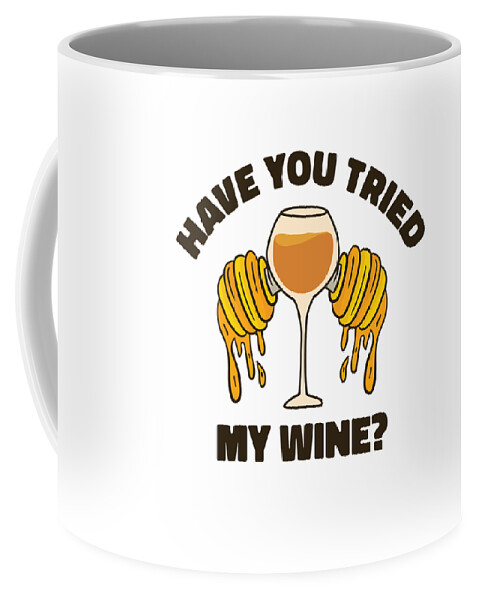The image depicts a simple white mug set against a white void background, with subtle shading to distinguish it from the backdrop. The interior of the mug is light gray, and it has a large handle positioned towards the back. On the front of the mug, in bold black all-caps text, the phrase "HAVE YOU TRIED MY WINE?" is displayed, with "HAVE YOU TRIED" arced above an illustration and "MY WINE" positioned straight below it. The central illustration features a wine glass filled with honey-colored liquid. On either side of the wine glass, there are two dripping honeycombs, adding a touch of whimsy to the design.